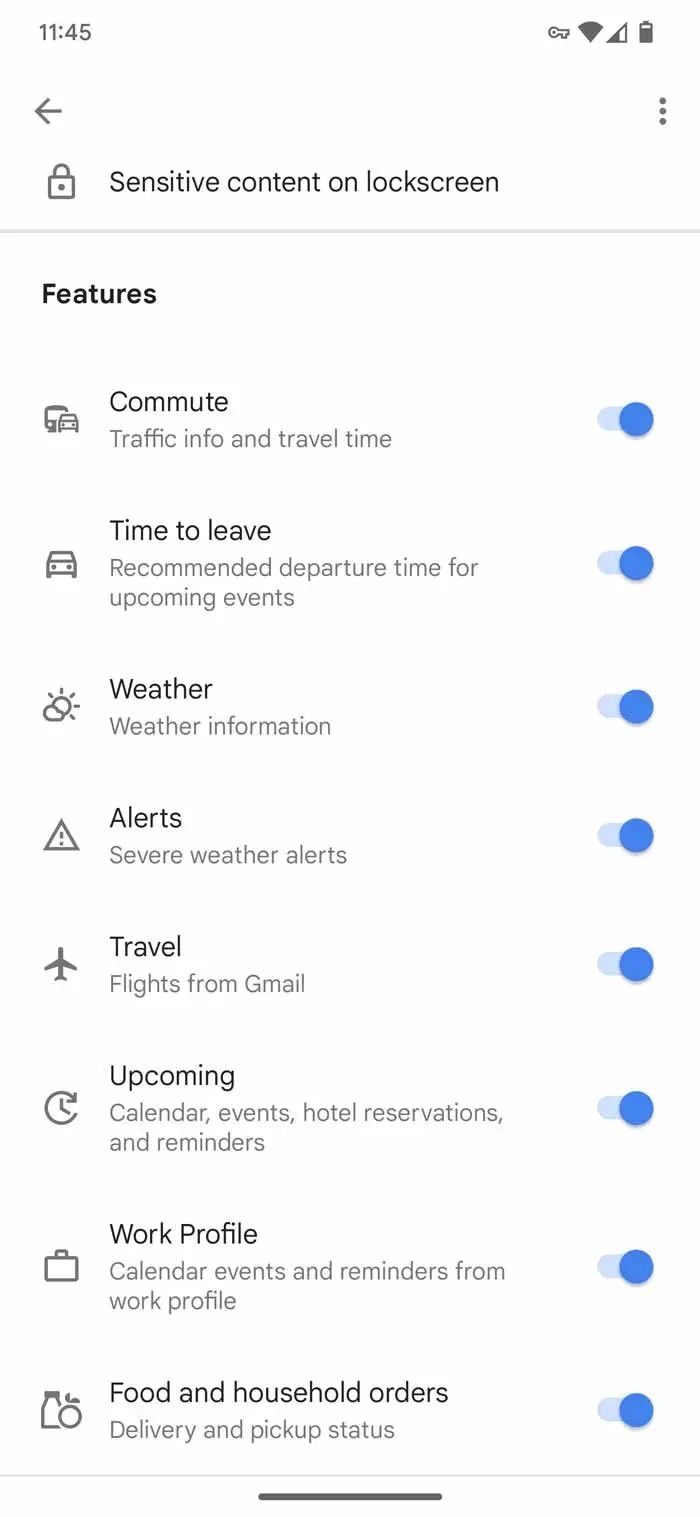The screenshot captured at 11:45 (time without a.m. or p.m. designation) displays a smartphone's settings menu under the "Sensitive Content on Lock Screen" category. 

**Top Status Bar:**
- Time: 11:45
- Wi-Fi signal indicator
- Weak cellular tower signal indicator
- Battery nearly full

**Menu Options:**
1. **Features:**
   - "Commute": Includes traffic info and travel time. The toggle switch is in the 'ON' position.
   - "Time to Leave": Recommends departure times for upcoming events. The toggle switch is in the 'ON' position.
   - "Weather": Provides weather information. The toggle switch is in the 'ON' position.
   - "Alerts": Sends severe weather alerts. The toggle switch is in the 'ON' position.
   - "Travel": Includes flight information from Gmail. The toggle switch is in the 'ON' position.
   - "Upcoming": Displays calendar events, hotel reservations, and reminders. The toggle switch is in the 'ON' position.
   - "Work Profile": Shows calendar events and reminders from work profile. The toggle switch is in the 'ON' position.
   - "Food and Household Orders": Provides information about orders. The toggle switch is in the 'ON' position.

The screenshot also includes a back button (arrow pointing left) on the bottom left and a three-dot menu icon on the bottom right, indicating additional options.